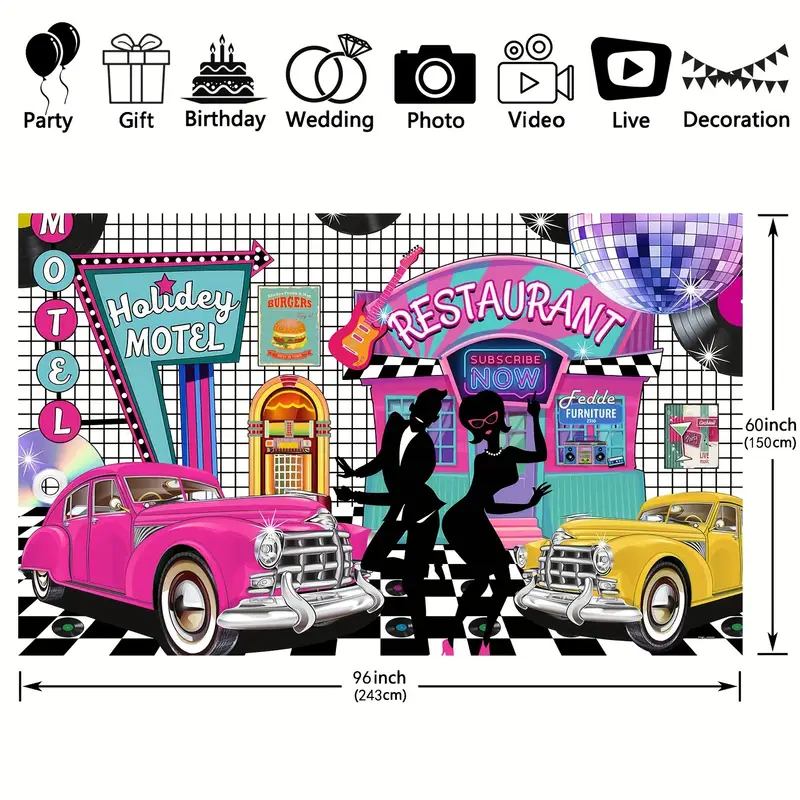This cartoonish and vibrant advertisement depicts a lively 1950s-themed party scene. At the top, black and white logos featuring balloons and a "Party" sign set a festive tone. Below, various symbols including birthday cakes, wedding rings, and cameras represent different celebration elements. Dominating the scene are two retro cars, one purplish-pink and the other gold, parked against a backdrop of neon signs and vintage decor. The scene is animated with silhouettes of a man in a suit and a woman in a dress dancing energetically on a checkerboard floor, surrounded by records and a jukebox. To the left, a "Holiday Motel" sign and a restaurant symbol contribute to the nostalgic ambiance. Measuring 60 inches vertically and 96 inches horizontally, this colorful poster employs a palette of blue, pink, orange, yellow, and various other hues, evoking a sense of joy and excitement associated with 1950s rock 'n' roll culture.